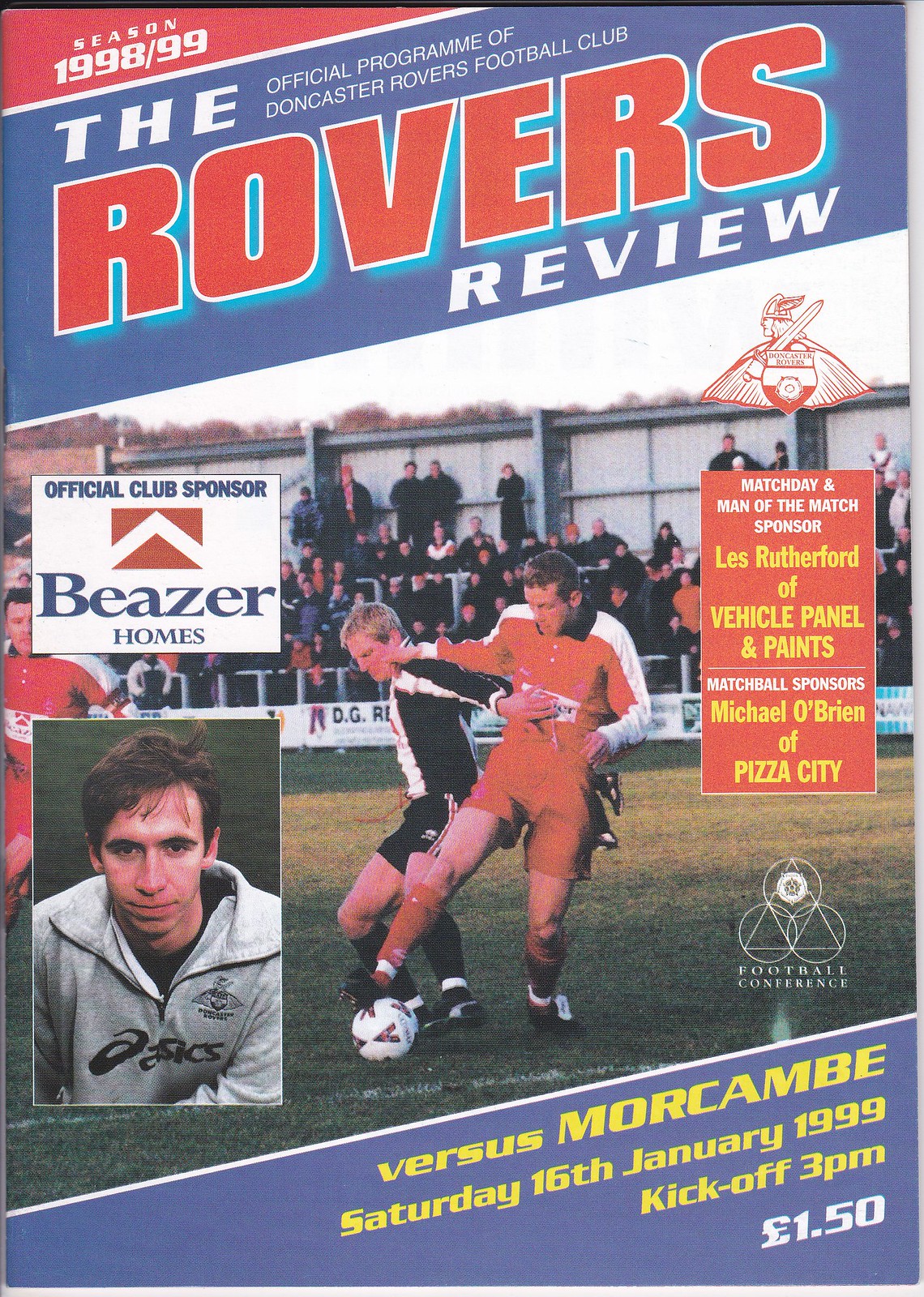The front cover of the Doncaster Rovers Football Club official program, titled "The Rovers Review" for the 1998-99 season, features a striking design with a blend of red, blue, black, and white colors. At the top-left corner, a red section indicates "Season 1998-99," followed by a diagonal blue banner that reads "THE" in large white capital letters, and underneath in smaller print, "Official Program of Doncaster Rovers Football Club." Dominating the cover, "ROVERS" is prominently displayed in large capital red letters with a 3D white outline and blue shadow, and "REVIEW" is beneath in large white letters.

Centered on the cover is an action photo of two soccer players: one in a red uniform, kicking a soccer ball, and the other in a black-and-white uniform, with their arms interlocked, fervently contesting for the ball on a grassy field. Spectators can be seen in the background, some standing and others seated in bleachers.

On the left side of the cover, there is a rectangular close-up of a young man with short brown hair, wearing a gray jacket. Above this image is an advertisement in a white square, stating "Official Club Sponsor" alongside the Beazer Homes logo.

On the right-hand side, a smaller image depicts a man in a hoodie. Accompanying this image is an orange box listing "Match Day and Man of the Match Sponsor: Les Rutherford of Vehicle Panel and Paints," and beneath it, "Match Ball Sponsors: Michael O'Brien of Pizza City". Along the bottom of the cover, a light blue diagonal banner displays in red letters, "Versus Morecambe" and in smaller text, "Saturday 16th January 1999, Kickoff 3 p.m., £1.50".

This detailed and visually engaging design serves as both a program and a promotional piece for the club's game against Morecambe.